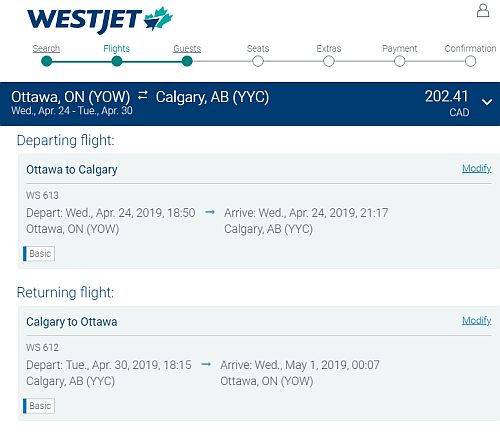This image depicts a webpage from the WestJet flight booking website. Prominently, the "WestJet" logo appears in blue at the top left corner, accompanied by the company's logo. Below it are navigation tabs labeled "Search Flights," "Guest Seats," "Extras," "Payments," and "Confirmation," indicating a user is navigating through the flight booking process. 

The user appears to be booking a round-trip flight from Ottawa, ON to Calgary, AB, scheduled from Wednesday, April 24th to Tuesday, April 30th. The total cost for this trip is $202.41 CAD. The webpage's aesthetic is dominated by blue, gray, white, and green colors. Additionally, there is an option to modify the booking before finalizing the payment. The overall design and functionality of the website are typical for booking flights.